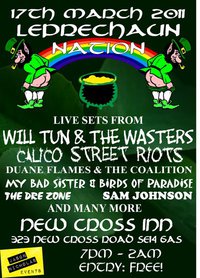This is a small digital image of a detailed festival poster for a St. Patrick's Day event. The background predominantly features shades of green and black, with a faded shamrock design. The header at the top, in white Gaelic script, announces "17th March 2011, Leprechaun Nation." Central to the design are cartoon depictions of leprechauns with their trousers pulled down, connected by a rainbow, with a pot of gold situated between them. Below, in clear white text, the poster lists musical acts including Will Tun and the Wasters, Calico Street Riots, Dwayne Flames and Coalition, My Bad Sister, Birds of Paradise, The Dre Zone, Sam Johnson, and many more. The event is scheduled to take place at New Cross Inn, located at 323 New Cross Road, SE14, with free entry from 7 p.m. to 2 a.m. The image also contains additional contact details and a yellow rectangle, likely displaying a logo or further information, although it is difficult to read due to the image's small size.